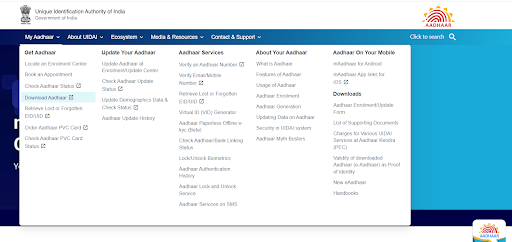This image showcases a webpage from the Unique Identification Authority of India (UIDAI). At the top left of the page, there is the UIDAI logo. The webpage itself features a blue background, but a large, predominantly white pop-up box occupies most of the screen. The only portion of the webpage background visible outside the pop-up is the menu bar, which runs across the top. 

Beneath this menu bar, the white pop-up box is divided into multiple sections organized in columns. From left to right, the sections are labeled "GET AADHAAR," "UPDATE YOUR AADHAAR," and "AADHAAR SERVICES." Additionally, there is a "Download" section available.

In the top right corner of the pop-up box, there is an AADHAAR logo, depicting a sun with red spirals and orange triangular rays. Positioned below this logo is a "click-to-search" text or button, presumably for navigating within the site.